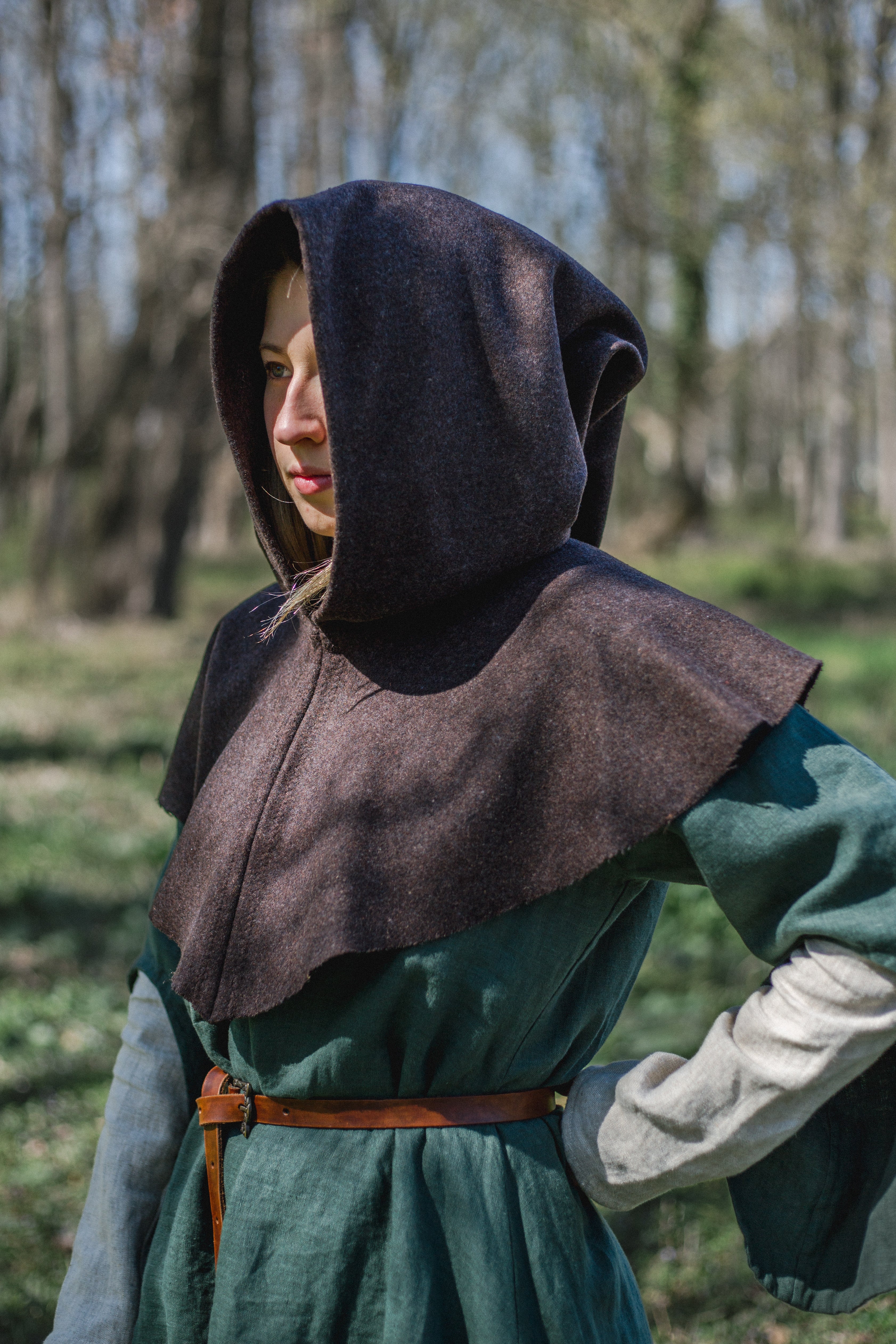The photograph captures a young woman standing in a sunlit, wooded area, surrounded by a field of grass and bare trees. She wears a distinct medieval-inspired outfit: a brown hooded dress over which a brown hood extends, partially covering her shoulders and chest. The bottom part of her dress is a mix of green and white, and she sports an orange leather belt tied around her waist. Her left hand rests on her hip while her right arm hangs down, out of sight. She is turned slightly diagonally, looking intently in front of her, with a tuft of blonde hair peeking out from under her hood. The natural sunlight enhances the scene, emphasizing the brightness and detail of the forest backdrop.